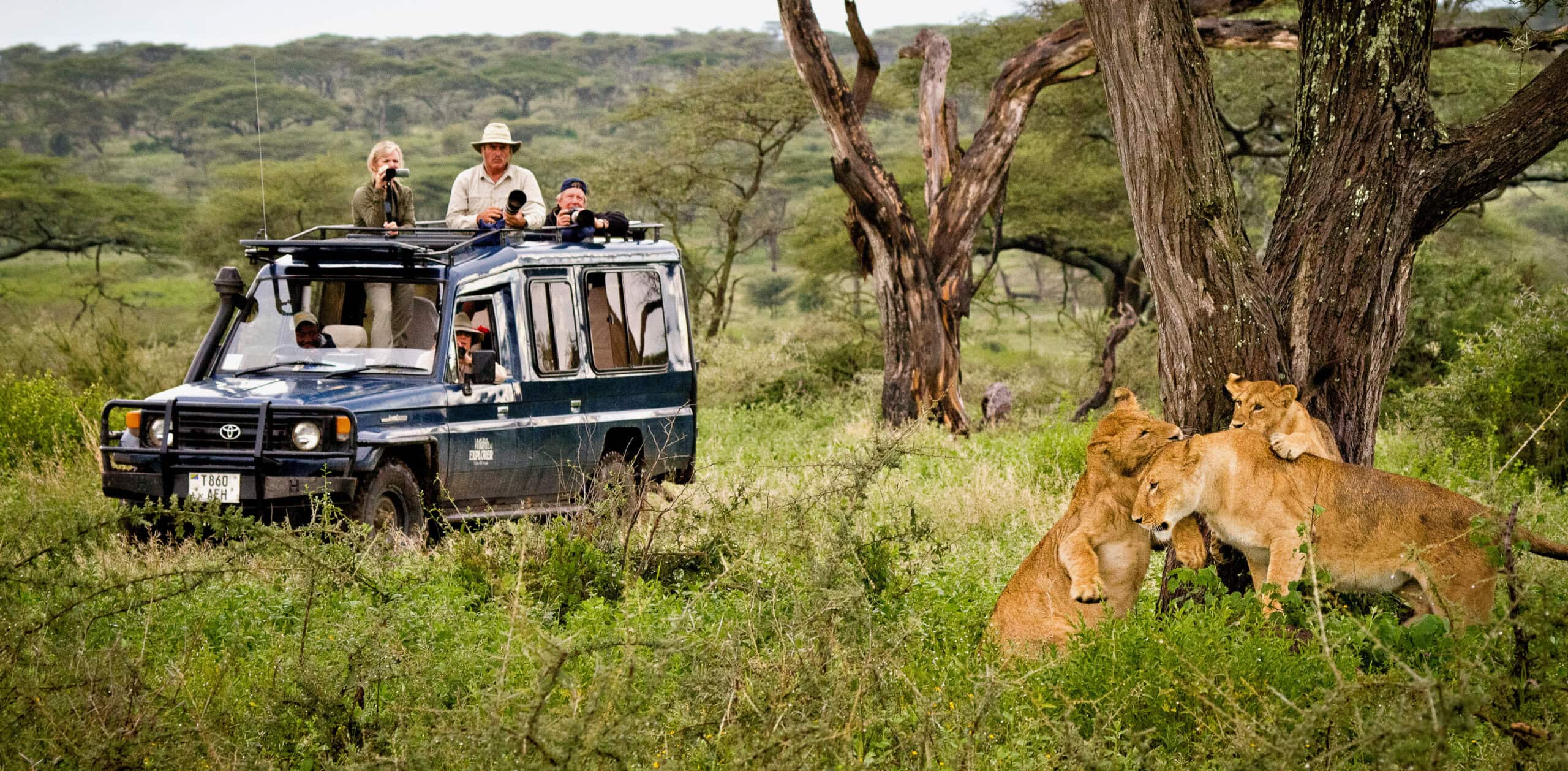This captivating photograph captures an African safari scene, featuring a blue Toyota safari vehicle with the license plate T860AFH and distinct radio antennas. The Toyota SUV has an open roof and large windows, allowing three tourists to stand up in the back, with two in the front seat. The tourists, equipped with cameras, are enthusiastically filming and photographing a mesmerizing group of lions. The focal point of the image is a female lion accompanied by her two nearly grown cubs. The majestic animals are situated near the trunk of a tree on the right side of the photograph, engaging playfully with each other. In the background, to the left of the image, the safari vehicle is positioned with its front facing the bottom left and its back towards the top right. Surrounding the scene are sparse bushes and the expansive wilderness of the African safari, with another tree and a rock slightly visible in the backdrop, highlighting the natural beauty and excitement of the safari adventure.